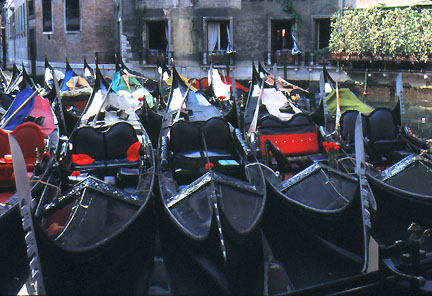The image is a high-contrast, surreal photograph featuring several canoes or gondolas aligned side by side in a row along a canal, likely in Europe. The canoes are predominantly dark grey or almost black, with some featuring red and black seating. The tips of the gondolas display varied colors such as blue, pink, white, and olive. The light illuminates the backs of the boats, creating a stark visual contrast against the predominantly dark bottom of the image. 

In the background, the photograph depicts the wall of an ancient, large greyish stone or brick building. The building appears to turn around a corner, showing a slightly browner tint towards the upper left-hand corner. Several large windows are visible, one of which seems to have a light on, while another has curtains. The upper right-hand corner of the image features a planter box or hedge with some light-colored vegetation, adding to the surreal ambiance of the scene.